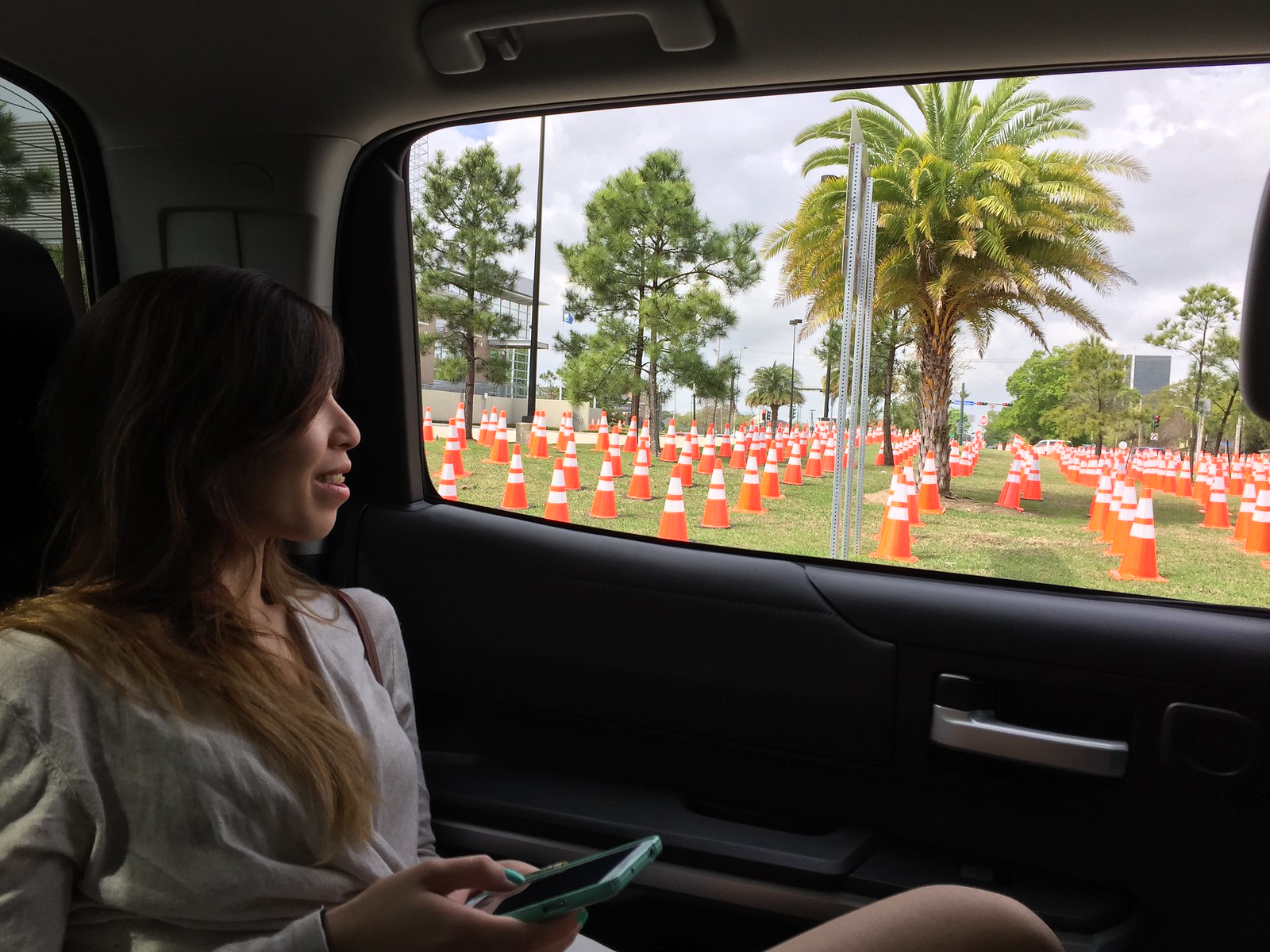A young girl looks out the window of a luxury car, her smile illuminated by the light from her cell phone that she holds in one hand. Outside, a surreal scene unfolds; a vast field stretches out, populated not with flowers or crops but with neat rows of bright orange traffic cones, each one topped with white reflective stripes. The sheer number of cones recedes into the distance, creating a striking visual that ends at a vanishing point, blending into an expanse of orange and white.

The tropical setting, complete with flourishing palm trees, adds a layer of irony to the image. The leather interior of the car, complete with a sizable handle and a luxurious finish, contrasts sharply with the peculiar outdoor scene. The girl's casual, almost lounging posture—with her legs crossed and seat tilted back—completes the whimsical nature of the photograph. The image invites multiple interpretations, from a commentary on no parking zones to an eerie resemblance to a graveyard where headstones have been replaced with pylons. It’s a humorous yet thought-provoking snapshot, capturing a moment rich in both visual and contextual irony.